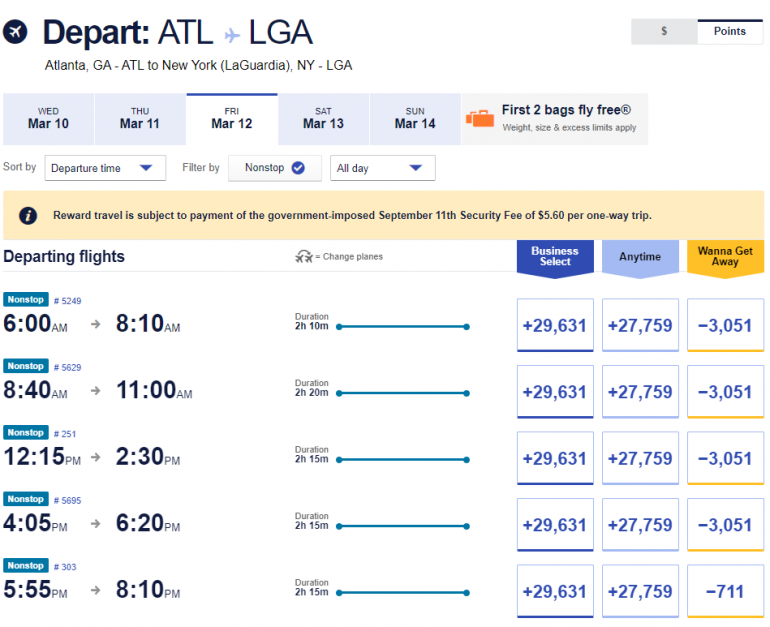At the top of the image, there is a small airplane symbol next to the text, "Depart ATL -> LGA." To the right of this, there's a box with a dollar sign, followed by text that says "Points."

Below the "Depart ATL" section, the text reads "Atlanta, GA (ATL) to New York, LaGuardia, NY (LGA)."

Underneath this, there are several boxes with dates: "Wednesday, March 10th; Thursday, March 11th; Friday, March 12th; Saturday, March 13th; Sunday, March 14th."

Next, there is a small orange suitcase symbol with the text, "First two bags fly free. Weight, size, and excess limits apply."

Following this, there are drop-down menus for sorting and filtering options. One drop-down reads "Sort by" with options like "Departure time," marked by a small airplane icon. Another drop-down reads "Filter by," with a checkbox next to "Non-stop," followed by options like "All day."

A yellow bar highlights important information: "Reward travel is subject to payment of the government- and post-September 11th security fee of $5.60 per one-way trip."

Below this, there's text that reads "Departing flights: Change planes. Business Select, Anytime, Wanna Get Away."

Further down, various flight options are displayed with details such as departure times, flight durations, and costs. There are five different flight options presented, each with varying departure times but similar durations and differing prices.